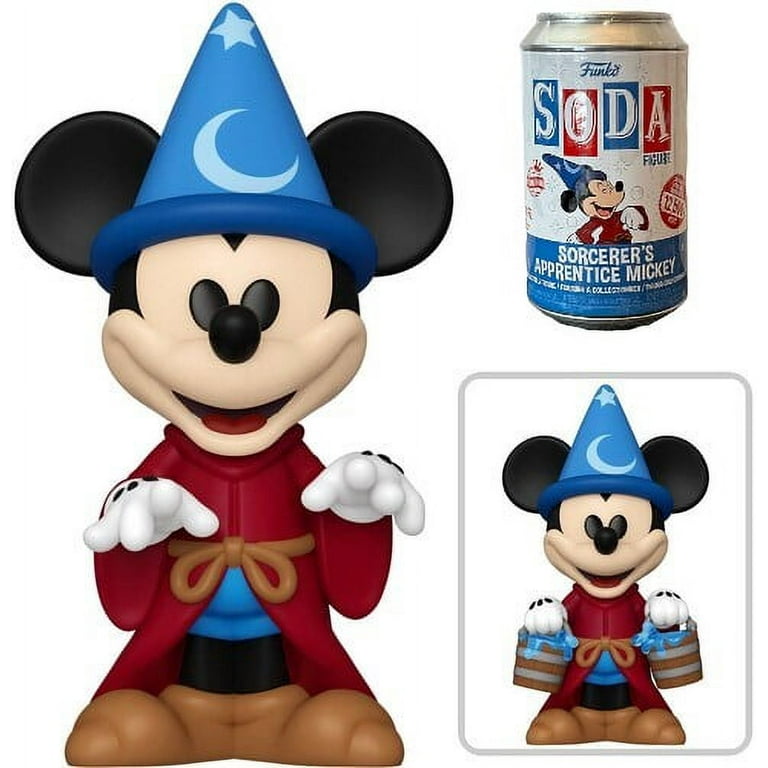This image is a detailed collection of Sorcerer's Apprentice Mickey Mouse-themed items from Walt Disney World. Featured prominently is Mickey Mouse in his iconic outfit from Fantasia, wearing a blue wizard hat adorned with a white crescent moon near the bottom and a white star at the top, and dressed in a red Sorcerer's Apprentice robe tied with a brown drawstring. Mickey is also wearing his signature white gloves, brown shoes, and black pants. 

There are three distinct objects in the image. On the left is a figurine of Mickey standing with a big smile and his hands raised as if about to perform magic. In the bottom right corner, a nearly identical figurine shows Mickey holding two wooden buckets overflowing with blue water, mirroring a classic scene from the movie. In the top right corner, there is a small, vintage-style silver soda can labeled "Funko Soda" featuring "Sorcerer's Apprentice Mickey" in the same iconic outfit. The label is red, white, and blue, and depicts Mickey marching across the can. Each item encapsulates the whimsical and enchanting essence of Mickey Mouse as the Sorcerer's Apprentice.